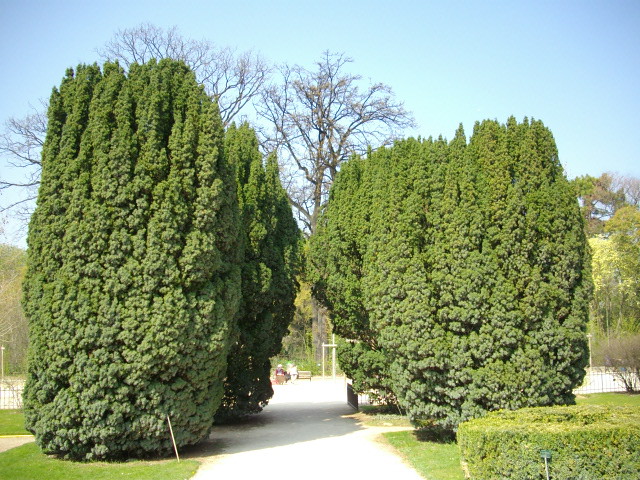In this bright daytime outdoor photo, the scene features an entrance to a garden or park framed by several distinctly tall and column-like bushes, which stand about 20 to 30 feet high. These striking shrubs, two on the left and at least two on the right, are carefully shaped with rounded sides and look somewhat like spiky hair standing straight up. The tall shrubs are lush and very green, contrasting with the leafless branches of taller trees in the background. In the lower right corner, there is a small, meticulously trimmed bush next to a small solar light. The walkway beside this bush leads into the park area, where small patches of green grass dot the area around the tall shrubs. Off in the distance, a man can be seen sitting on a bench, surrounded by the overall greenery and the clear blue sky above, which adds to the serene ambiance of this well-maintained outdoor space.